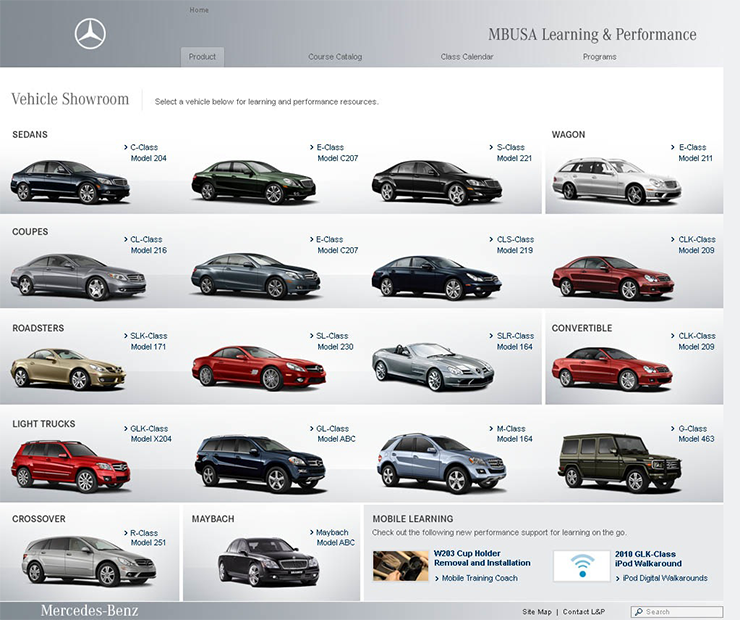Caption: 

The Vehicle Showroom on the Mercedes website showcases an extensive array of high-end vehicles arranged in five distinct rows. The top row is dedicated to sedans, followed by coupes, roadsters, light trucks, and crossovers. In the crossovers section, there are only two vehicles displayed, while all other categories feature four models each. Among the vehicles, there is a notable convertible and a station wagon, adding variety to the display of luxurious Mercedes cars. The roadster stands out as a sleek sports car, epitomizing elegance and performance. The predominant colors of the cars are red, black, and silver, which complement the overall premium aesthetic of the main webpage, characterized by white and deep silver tones. At the bottom of the page, a distinguished black Maybach is visible, which, although unpriced, undoubtedly reflects an exceptional level of luxury and exclusivity.